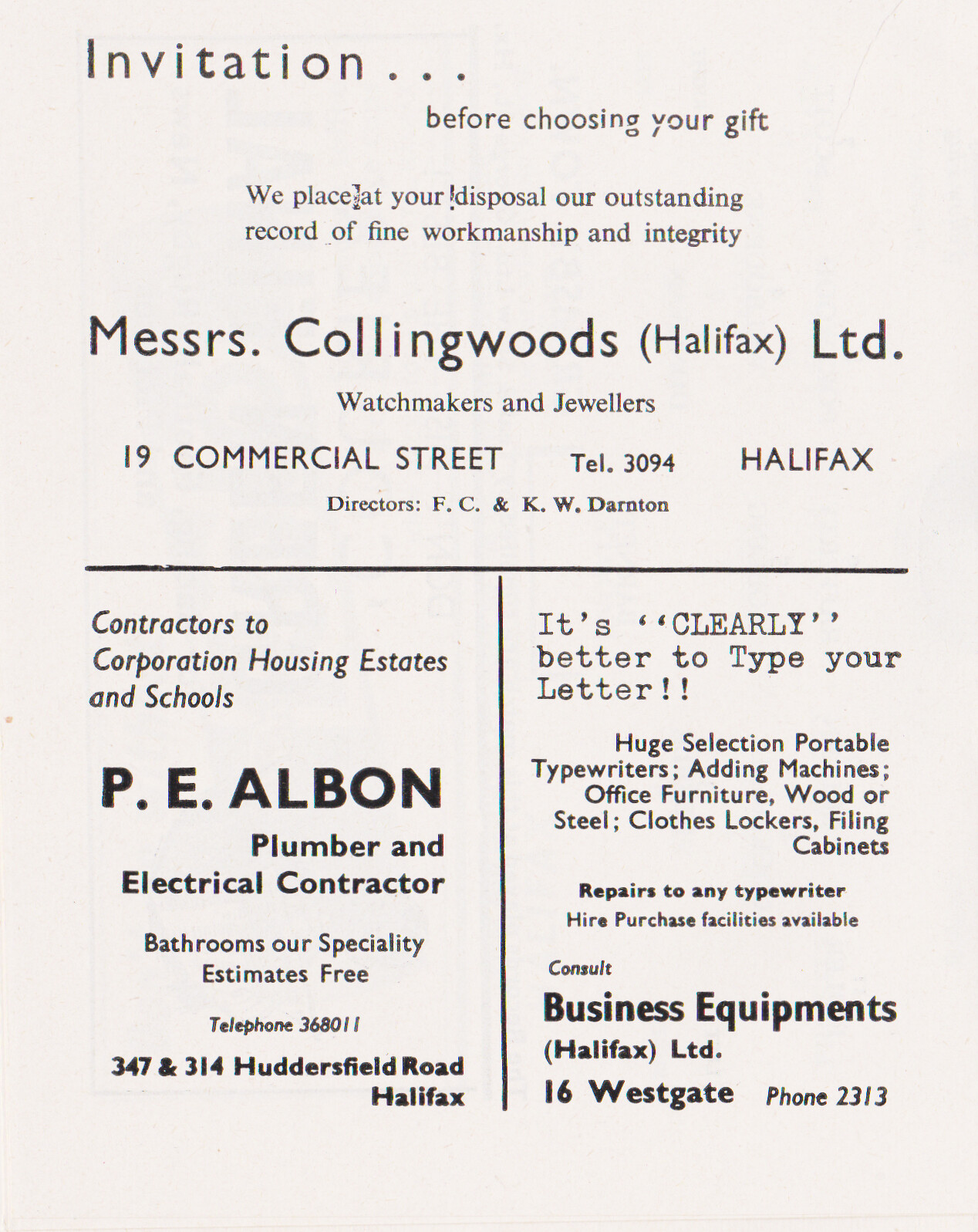An image displays an elegantly structured vintage advertisement, primarily divided into three distinct sections. The top section showcases a sophisticated text ad prominently featuring an inviting message: "Invitation." It extends an offer to potential customers, emphasizing the company's stellar reputation for fine workmanship and integrity. The ad proudly displays the name of the business, "Monsieurs Collingsworth Limited," specializing in watchmaking and jewelry. The company's address is listed as "19 Commercial Street," along with a contact telephone number, "309," in Halifax.

Below the main ad, the lower section is bifurcated into two separate advertisements. On the left, there is an ad for "P.E. Albon, Plumber and Electrical Contractor," with a bold statement: "Bathrooms are our specialty." The ad assures prospective clients that estimates are provided free of charge.

The right section presents an ad with a clear and persuasive message: "It's clearly better to type your letter." This ad promotes a wide range of office supplies including portable typewriters, adding machines, office furniture in both wood and steel, clothes lockers, and filing cabinets. Additionally, it offers repair services for any typewriter, encouraging potential customers to consult "Business Equipments" in Halifax for their office needs.